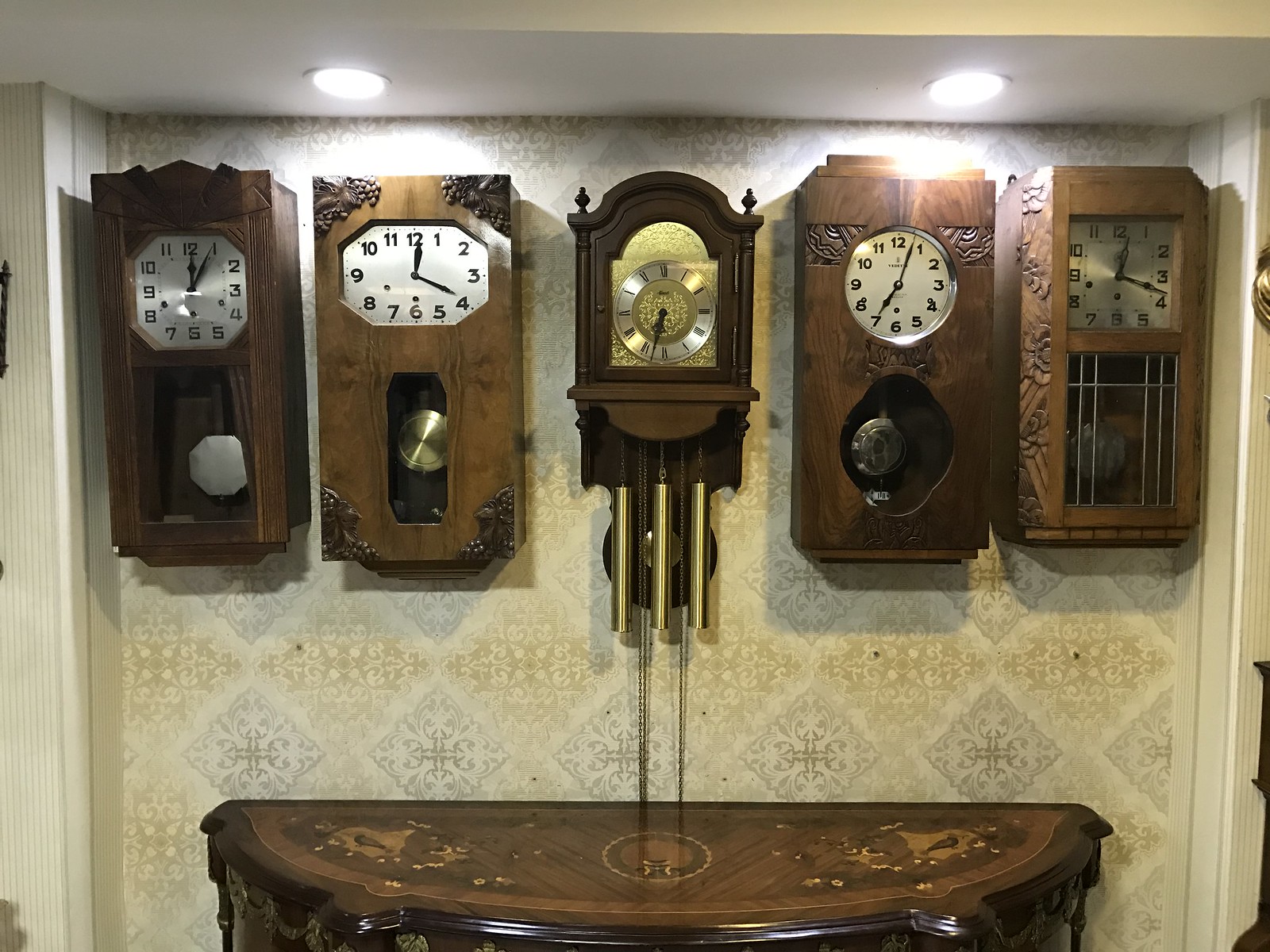This landscape photograph captures a color image of the interior wall of what appears to be a home, adorned with five ornate wall-mounted clocks. Each clock, modeled in a short grandfather style, is framed with intricately carved wooden borders, which vary from dark mahogany to lighter brown tones. The central clock stands out with its more elaborate design, featuring three bell tubes and additional hanging weights beneath its metallic clock face. These clocks are not supported by any furniture and appear to be affixed directly to the wall, which is covered with vintage wallpaper decorated with diamond patterns and ornate detailing.

Beneath the clocks sits an elegant, dark brown half-circle table, its flat edge flush against the wall. The table is polished to a shine and embellished with scenic carvings. The scene is illuminated by two recessed ceiling lights that cast a whitish glow over the ornate wall and table below, adding a warm ambiance to the room that resembles a cozy, well-kept home.